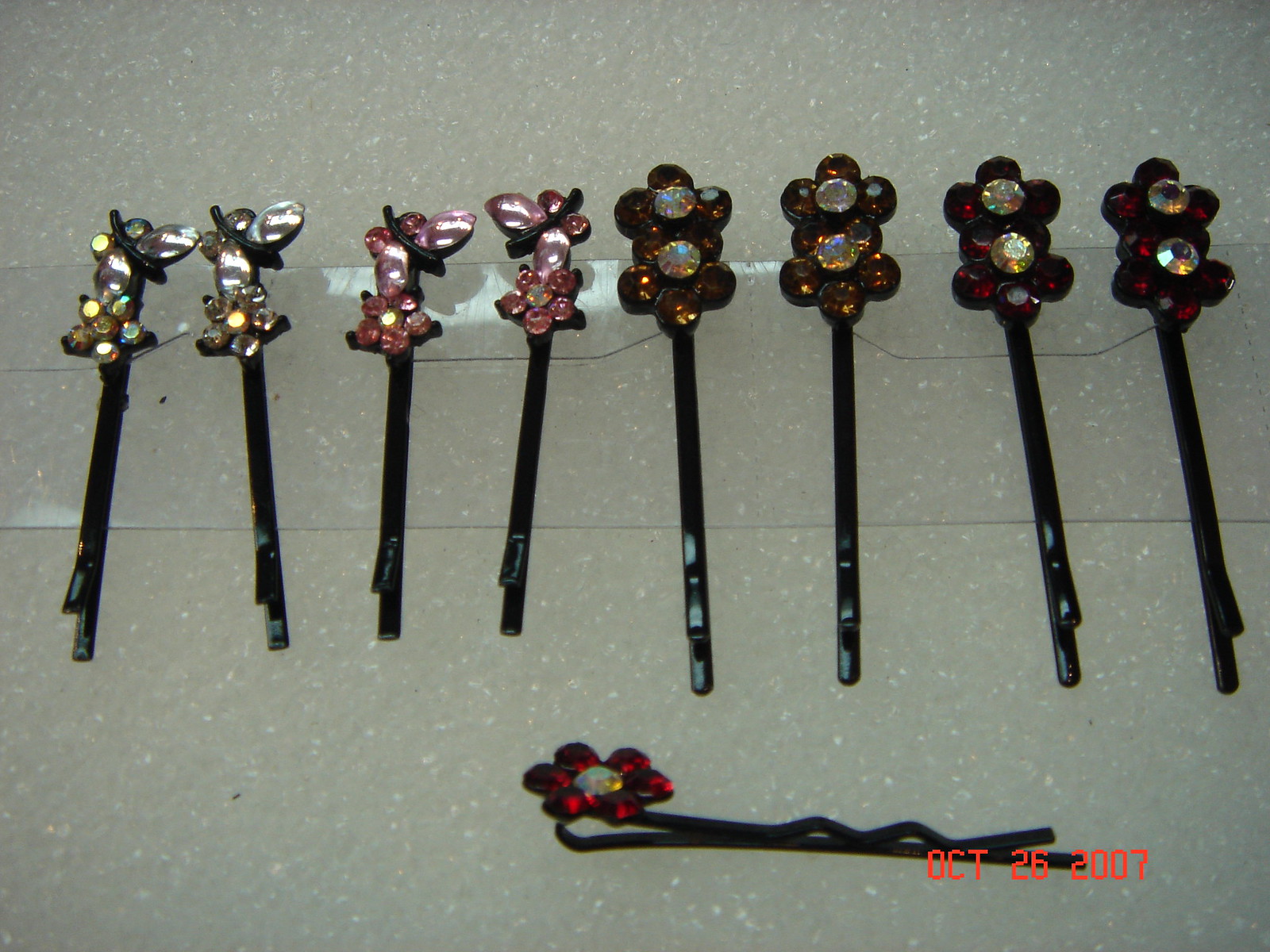The image is a photograph of nine intricately designed black bobby pin clips, each adorned with six-petaled flower decorations. These flowers sparkle with gemstones in a range of colors—pink, white, yellow, amber, ruby, and a prism-like shimmer, with lighter diamond-like centers. The clips are affixed to a rectangular plastic sheet and positioned against a light grayish, sparkly marbled countertop. Eight of the clips are arranged vertically in pairs, with color sequences from left to right being gold, pink, dark orange, and dark red. An additional bright red flower clip lies horizontally below these pairs. At the bottom right corner of the image, a red date stamp reads "OCT 26 2007," marking the photograph's date.